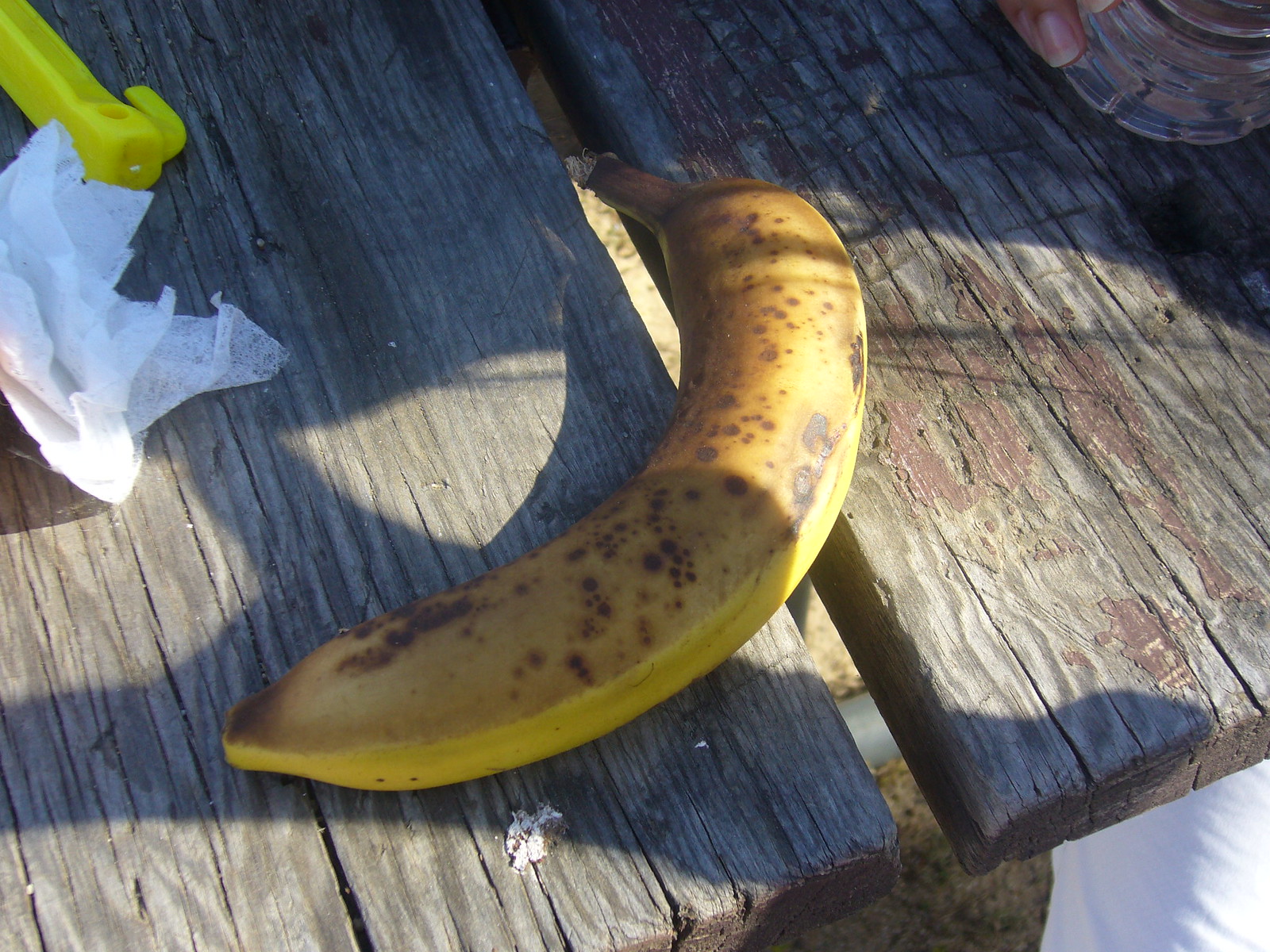A close-up image captures the detailed texture and aging character of a rustic, gray wooden table with noticeable cracks along its grain. Remnants of a brown varnish on the right side reveal the table's vintage quality. In the upper right, a white crystal-like glass cup is held by a fingernail, adding a human element to the scene. Dominating the center, a large, vividly ripe banana rests on the table's edge. The banana's yellow skin is heavily speckled with numerous brown spots, indicating its advanced ripeness. In the upper left corner, a small piece of white paper towel and a yellow object add subtle detail to this richly textured and organically composed scene.